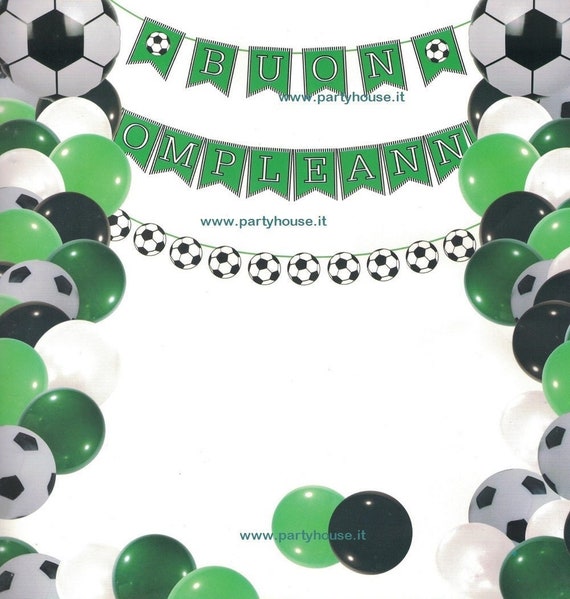This is an advertisement for an Italian party supply business called PartyHouse.it, specializing in fun get-together essentials. The image features a festive theme with a combination of black, white, and green colors. On the top corners and down the sides, there are decorations including balloons in light green, dark green, black, and white, as well as classic black and white soccer balls. Along the bottom, additional soccer balls and green balloons are displayed. 

Centrally, slightly above the middle, there's a green curved line, resembling a smile, adorned with soccer ball shapes, totaling around 10 or 11. Three horizontal lines run across the image, reminiscent of string banners, each contributing to the festive look. The topmost line features individual green flags with white letters spelling "BUON," interspersed with soccer ball flags. Below that, another string banner reads "COMPLEANNO," though it appears slightly jumbled as "OMPLEAN" in parts, clearly intending the Italian word for "Happy Birthday."

Moreover, the website "www.partyhouse.it" is prominently displayed in light blue text in three different locations: near the top, above the middle, and near the bottom of the image. This inclusion identifies the card as associated with an Italian company providing party supplies. The overall background of the image is white, enhancing the visibility of the decorations and text, making it a vivid and inviting advertisement for a festive product range.